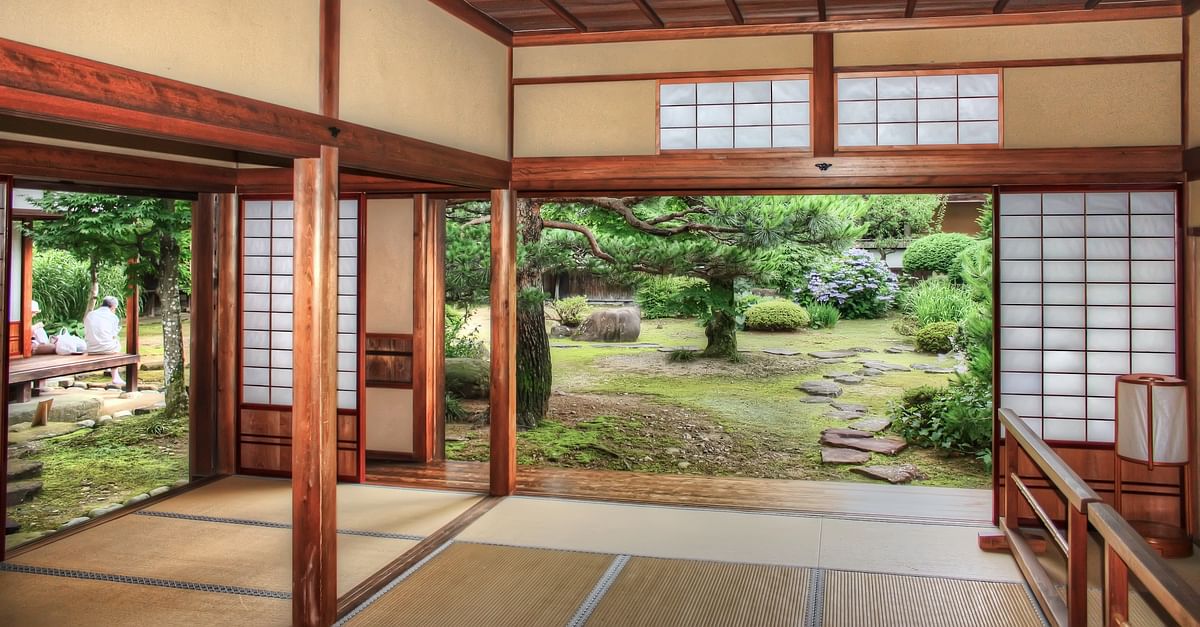This image captures the serene interior of a Japanese home or possibly a resort. The prominent feature is the bamboo flooring, segmented by darker tan and light tan shades, which adds a warm, inviting ambiance to the space. The walls and ceiling are supported by beams made of dark brown mahogany wood. Large sliding doors, constructed from a combination of wood and paper with white rectangular grids, open out to reveal a meticulously manicured garden. The garden is adorned with granite stone pathways and an array of lush, well-kept shrubs and trees, including a pine tree. On the left side of the image, an older man sits on a bench, gazing thoughtfully at the tranquil garden. The house itself is minimalistic, with no visible furniture other than the bench, emphasizing the clean and uncluttered Japanese aesthetic. The sky is overcast, casting a gentle, diffused light over the serene scene.